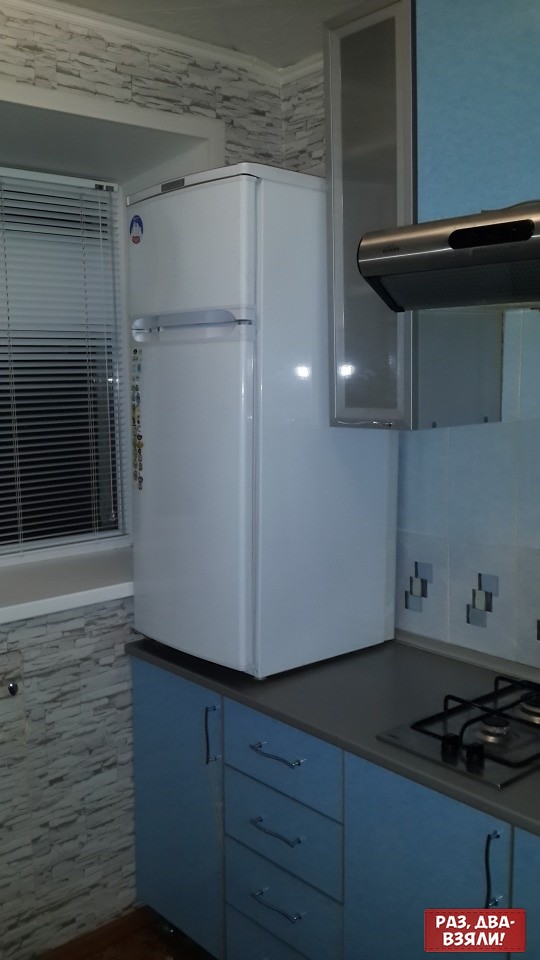The image depicts a detailed corner of a kitchen featuring a prominent white refrigerator with a freezer section on top, placed uniquely on a gray countertop. This refrigerator, resembling one suitable for an apartment and slightly larger than a mini fridge, is adorned with stickers and has a silver handle. It sits against a backsplash of intricately designed wallpaper made to look like stone. Below the refrigerator, blue cabinetry with long chrome handles lines the bottom, providing a striking contrast to the silver appliances and gray countertop. To the right of the refrigerator is a gas stove, topped with a stainless steel range hood. A nearby window, partially covered by a window shade, adds natural light to the setting, complementing the kitchen's cozy yet functional layout. Additionally, written in the lower right corner of the image, there is white text on a red background, possibly in Russian or a related Cyrillic script, lending an international touch to the scene. The photograph appears to be taken at nighttime, adding a warm, homey ambiance to the image.